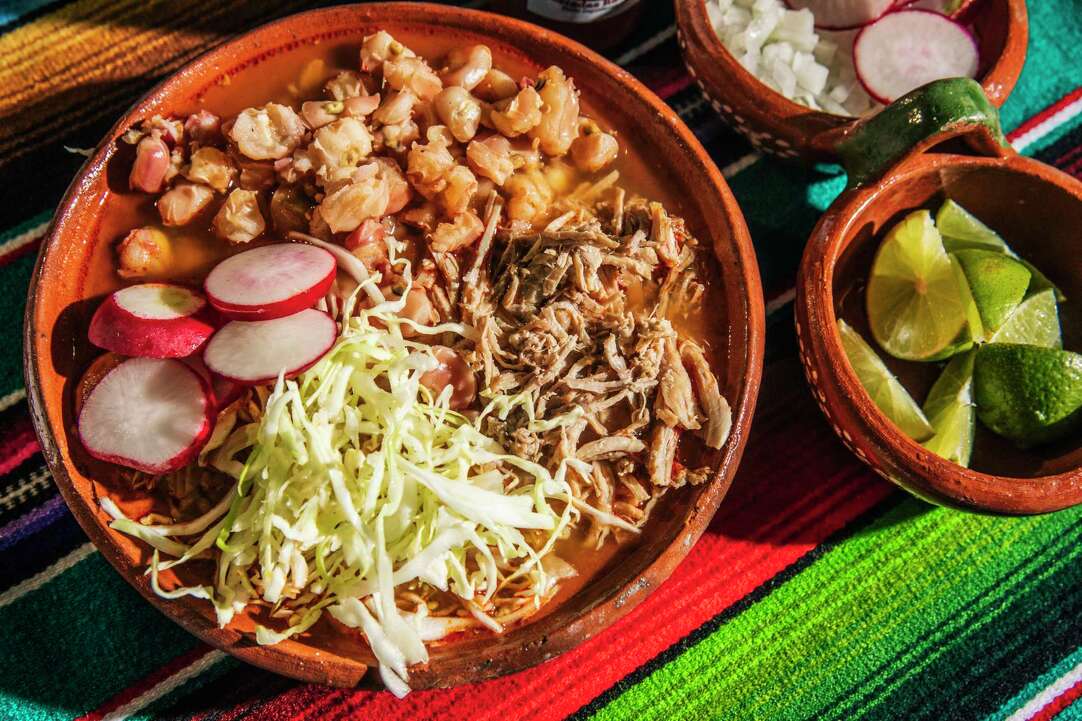The image is a brightly colored photograph, likely taken in direct sunlight, showcasing a vibrant and inviting Mexican meal. Central to the composition is a large, dark-colored wooden or pottery clay bowl nearly filling the top and bottom left side of the image. This bowl contains a rich, dark broth soup garnished with shredded lettuce or cabbage, pulled chicken or pork, sliced radishes, and another golden tan vegetable. To the right of this central bowl is a smaller clay bowl filled with fresh lime wedges. Just above the lime bowl is a half-visible small bowl containing chopped onions and additional sliced radishes. All of these bowls are artfully arranged on a diagonally patterned Mexican fabric blanket, featuring an array of bright colors such as yellow, brown, black, white, purple, red, and green. The diagonal placement of the blanket's pattern adds a sense of movement, drawing the eye to the delicious-looking food at the center.